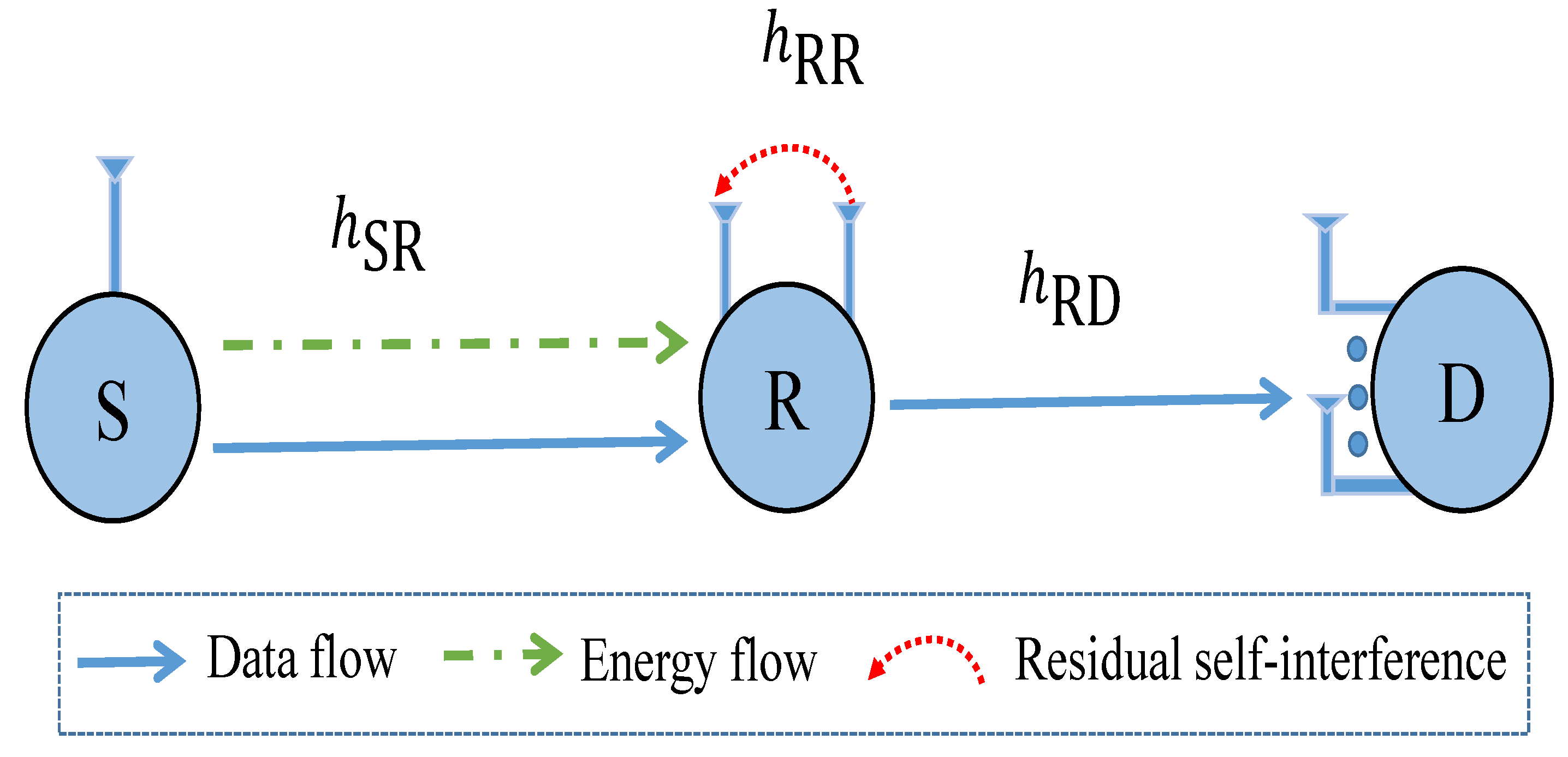In this detailed schematic illustration, we observe a graph and a chart depicting data flow (blue arrows), energy flow (green arrows), and residual self-interference (red arrows) between three points labeled as S, R, and D. The blue data flow arrow originates from S, marked within a circular bubble, and extends rightward toward R. Alongside this blue data arrow, a green dashed arrow signifies energy flow also extending from S to R. Above this section, the label "HSR" is prominently displayed. Further, a red arrow representing residual self-interference (HRR) extends between two points within the R section, symbolizing interference from the right to the left side of R. Lastly, from R, a continuous blue data flow arrow proceeds towards D, under the heading "HRD", illustrating the final data transfer within the chart.